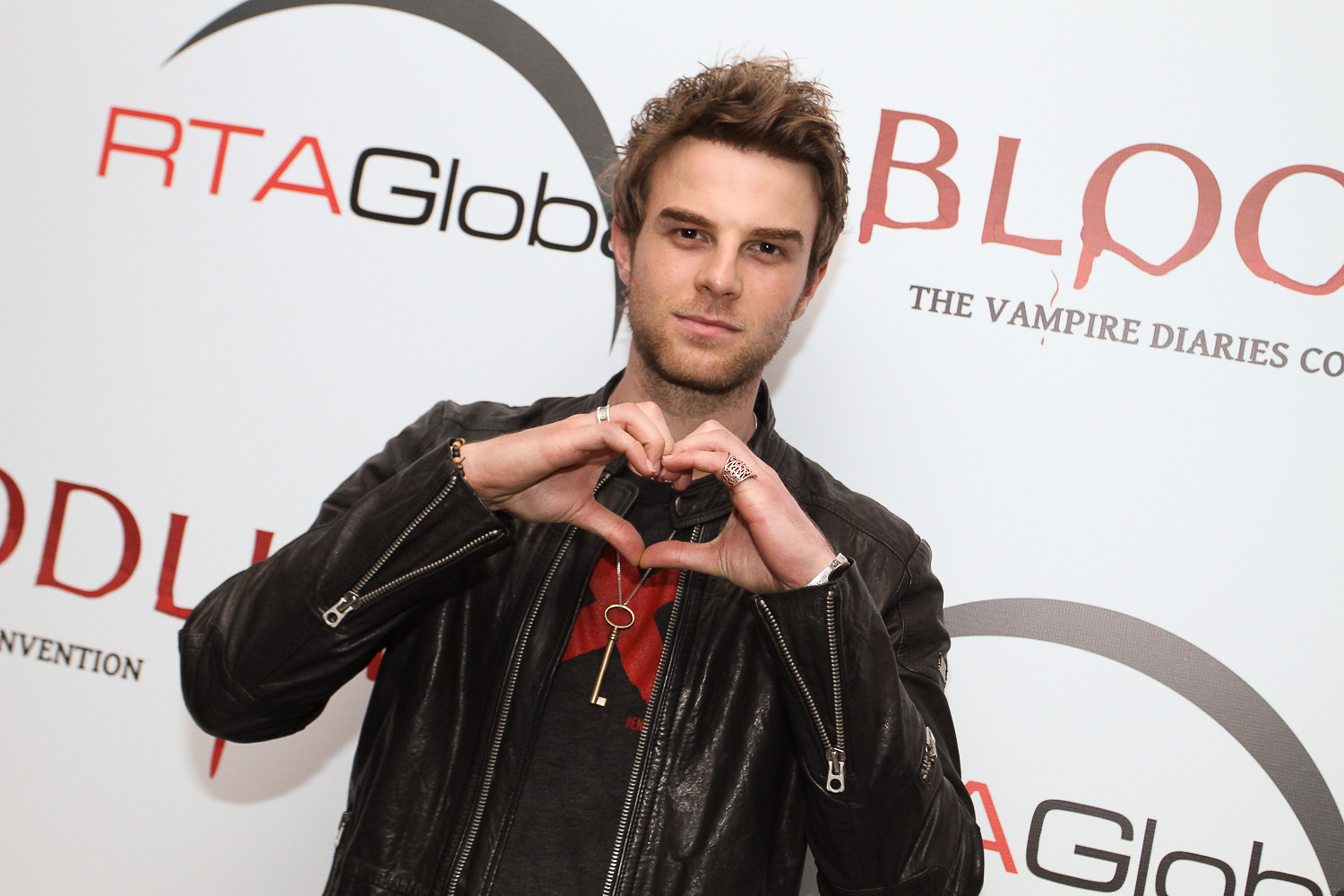A young, good-looking man with fair skin and brown, messy gelled hair stands slightly tilted to the right in front of a whiteboard backdrop. He’s wearing a black leather jacket with open zippers on the cuffs and front, and a black graphic t-shirt featuring a red "X" design. Around his neck, he has a chain necklace adorned with an old-fashioned gold key. He forms a heart shape with his hands right in front of his neck and wears silver rings. The backdrop behind him has repeated logos: on the left, “RTA” in red font followed by “Globe” in black font, with a curved line cutting through the "E" in “Globe” and circling back to the "R" in “RTA”; on the right, in a blood-dripping red font, it reads “Bloodlines. Below that, it says “The Vampire Diaries Convention.” The backdrop and the setting suggest a promotional event or photo op, likely for The Vampire Diaries Convention. The man's smoldering smirk and the overall setting give an impression of a professionally staged photograph.